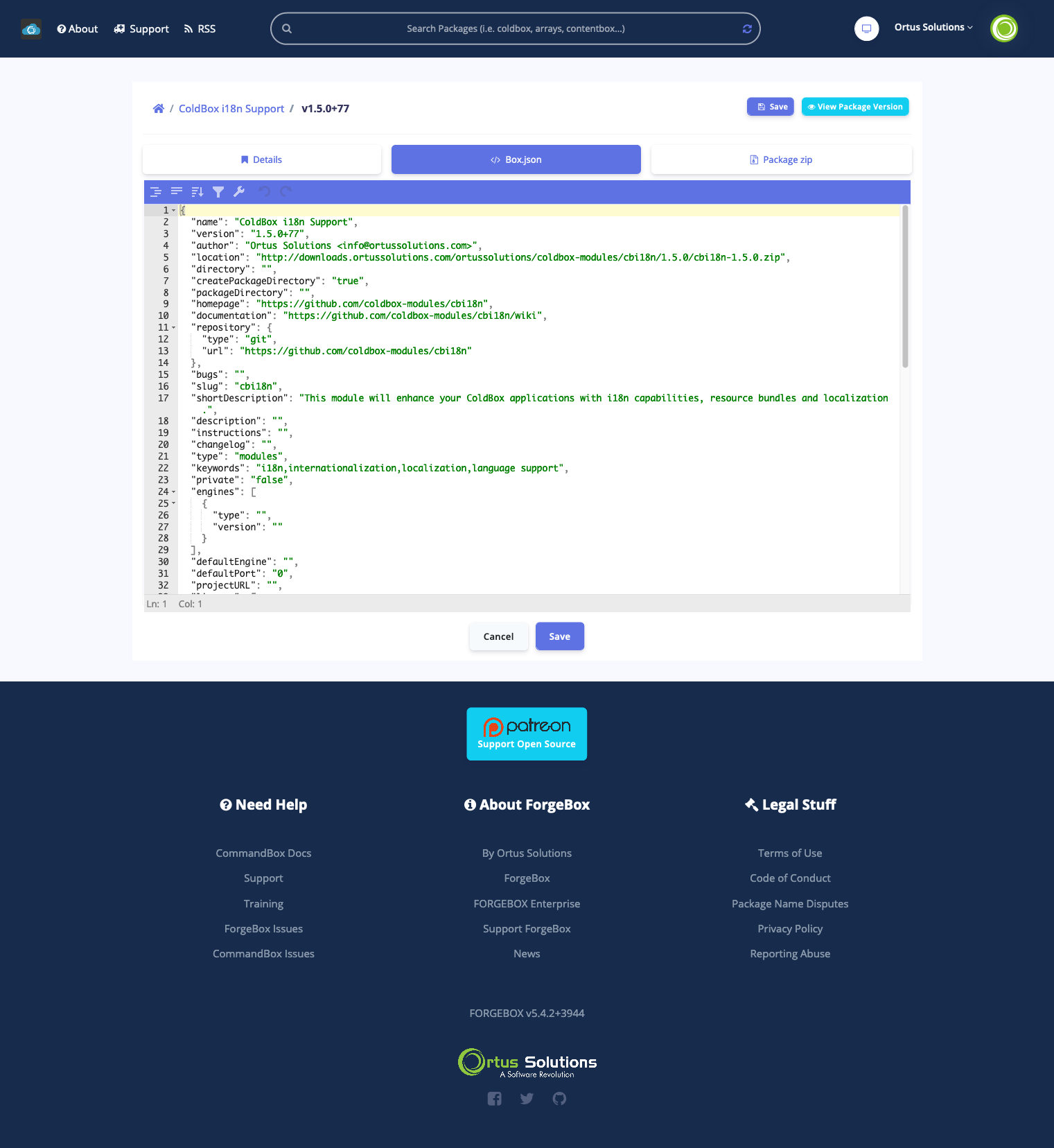The image features a predominantly white background with several key elements organized in a structured layout. 

At the top of the image, there is a dark blue rectangular box. Inside this box, on the left side, there is a small blue cloud icon next to the word "Support." Various dotted lines or elements are also present in this area. To the right of this, there's a search button.

Below this section, a white circle containing what appears to be a small screen is surrounded by additional dotted elements and circles. One of these circles has a small green figure inside.

In the main body of the image, a small blue house icon is visible alongside blue text and buttons. These buttons vary in shade from dark blue to very light blue, interspersed with white buttons that have blue text. Continuing downward, there's a blue box with five small icons aligned horizontally at the top. 

Adjacent to these icons, on the left side of the box, there is a light blue numbered list ranging from 1 to 38, accompanied by text including the name "Calico support" and the word "Stop." Various answers or responses in green text are also visible here. To the right, a blue slide button can be seen.

Near the bottom of the image, another blue box appears with lighter blue elements labeled "LT1" and "CC1." Buttons marked "Cancel" and "Save" (in blue) are present here. 

The lower portion of the image contains a large dark blue box, which includes a lighter section at the top featuring a red "P" logo and the word "Patreon." Beneath this, terms like "Support down" and "Need help" in white text are visible, along with references to "Forgebox" and legal disclaimers. The bottom-most part of the image has the text "Ortis Solutions" with "Ortis" highlighted in yellow.